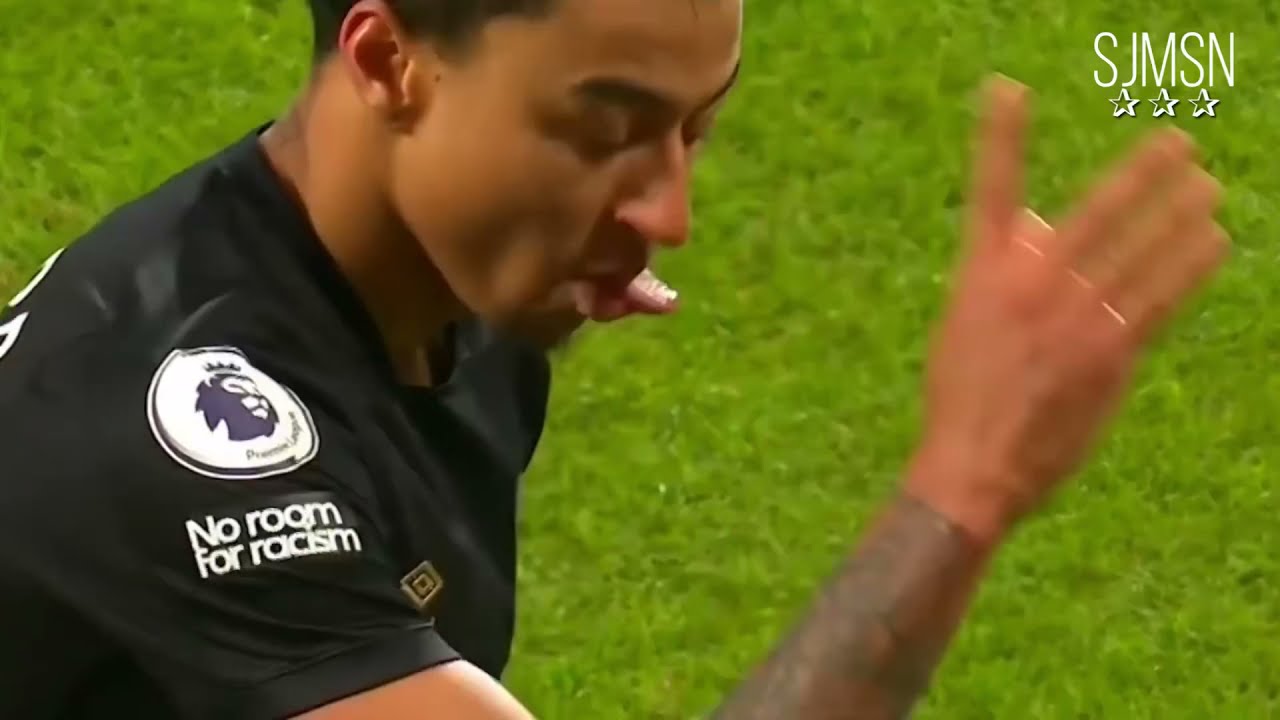In this photograph, a man is positioned against a backdrop of thick, green grass. The image features primarily his upper body, from his right shoulder upwards, as well as his right hand in the foreground, which appears blurred due to motion. The man wears a black, short-sleeved shirt adorned with a circular patch on his right shoulder. The patch features the outline of a lion with a crown, and beneath it, the white text reads, "No Room for Racism." 

His complexion is of a medium coffee tone with dark, short hair and matching dark eyebrows. Unique features include a freckle next to his ear on the left side and what seems like his tongue sticking out or possibly something ambiguous near his mouth. He appears to have some sort of glove, tattoo, or paint on his right hand, differing in color from his arm, adding to the image's initial confusion. His eyes are closed, and the motion of his arm conveys a dynamic moment captured. In the upper right-hand corner of the image, the white text "SJMSN" appears, followed by three stars. Overall, the photograph captures an intensely expressive moment set against a strikingly simple yet vivid natural backdrop.